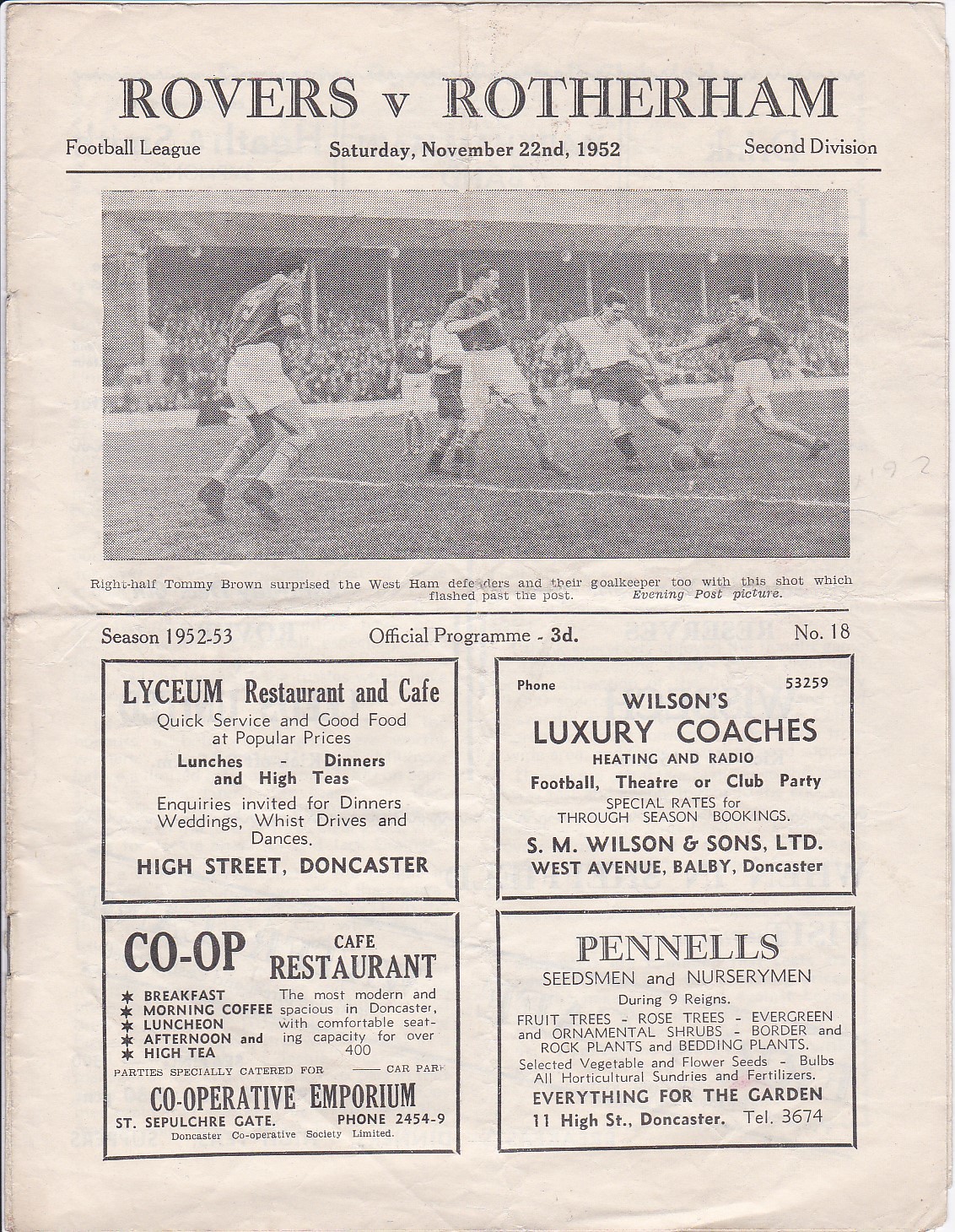This detailed vintage newspaper clipping or program page, yellowed with age, captures the essence of a historic soccer match between Rovers and Rotherham on November 22, 1952. The headline, "Rovers versus Rotherham, Football League, Saturday, November 22, 1952, Second Division," is prominent at the top. The entire page is in black and white, including a nostalgic image of the match. In the photograph, players from opposing teams—one team in white shirts and dark shorts, the other in dark shirts and white shorts—are captured mid-play, with the ball being contested and the goalie positioned to the left. Behind the players, a crowd of spectators fills the stands.

Beneath the image, the caption reads: "Right half Tommy Brown surprised the West Ham defenders and their goalkeeper with this shot which flashed past the post (Evening Post picture)." Further down, text indicates details such as "season 1952 to 1953," "official program 3d," and "number 18."

The bottom section of the page features advertisements for local Doncaster businesses:

- **Lyceum Restaurant and Cafe**: Quick service and good food at popular prices, offering lunches, dinners, and high teas. Located at High Street, Doncaster.
- **Wilson's Luxury Coaches**: Providing coach services for various events with special rates for through-season bookings. Operated by S&M Wilson and Sons Limited, Doncaster.
- **Co-op Cafe Restaurant**: The most modern and spacious in Doncaster, seating over 400 people. Services include breakfast, morning coffee, luncheon, afternoon and high tea, and party catering. Located at Cooperative Emporium, St. Sepulchre Gate, Doncaster.
- **Pennell's Seedsmen and Nurserymen**: Offering a range of garden essentials including fruit trees, rose trees, shrubs, and various seeds and fertilizers. Located at 11 High Street, Doncaster. 

This page serves not only as a program for a memorable soccer event but also as a charming piece of local history with business advertisements offering a glimpse into the past of Doncaster’s community.